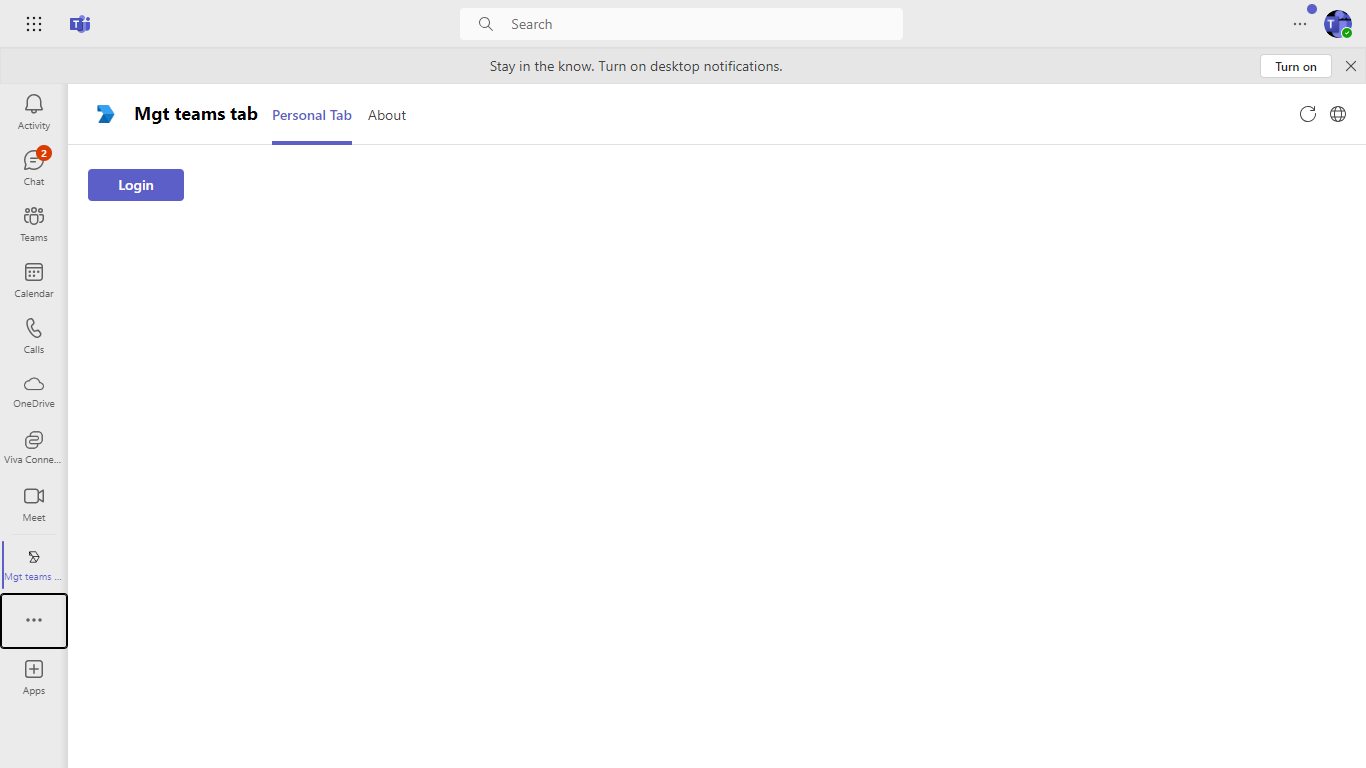The image depicts a screenshot of a web application interface, showcasing several distinct elements arranged in a structured layout. The outer border of the interface, including the upper and vertical tabs, is shaded in a light grayish blue tone. At the top of the interface, a horizontal rectangular tab is displayed, featuring nine tiny dots aligned on the upper left side. Adjacent to these dots is a blue "T" icon accompanied by two small people icons. Centrally positioned in this tab is a white search bar, beneath which the text "Stay in the know, turn on desktop notifications" is clearly visible, indicating that the interface is intended for a desktop environment rather than a mobile device.

Along the left-hand side, a vertical navigation pane lists several options in a column format. These options are labeled as follows: "Activity," "Chat" with a red circle displaying the number two, "Teams," "Calendar," "Calls," "OneDrive," "Viva Connection," "Meet," "Management Teams" (highlighted in blue), an icon represented by three dots enclosed in a black square, and "Apps" indicated by a plus sign within a square.

Dominating the center of the interface is a large white area divided into sections titled "Management Teams Tab," "Personal Tab," and "About." The "Personal Tab" is highlighted in blue, signifying the current active tab, while "About" remains in black. Beneath these tabs, a small rectangular blue button labeled "Login" in white stands out. There is no additional text present in this central section, maintaining a clean and uncluttered appearance.